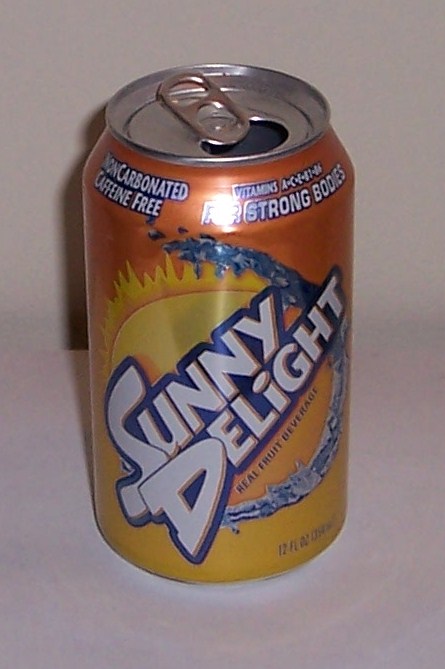In the image, a can of Sunny Delight is prominently featured, resting on a gray tabletop or countertop. The can transitions from a deep orange at the top to a bright yellow at the bottom, creating a gradient effect. The top left corner of the can displays "Non-Carbonated, Caffeine-Free" in white letters, surrounded by blue lines. This section also lists the vitamins it contains—A, C, E, B12, B2, and B6—highlighting its health benefits. Below this, there's a water design in a reverse C shape, curving down to the right. The brand name "Sunny Delight" is prominently displayed in white text against a blue background, accompanied by the phrase "A Real Fruit Beverage" in blue text. The top of the can is silver and is already opened.